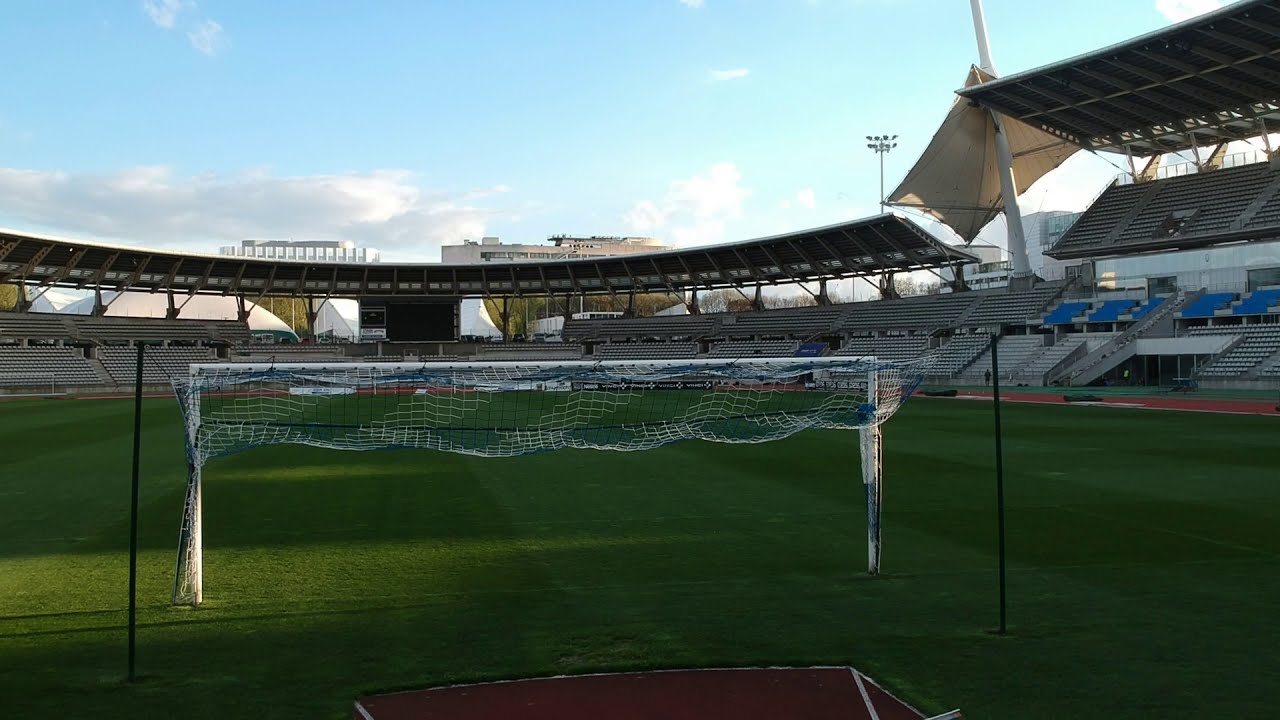This color photograph, taken from behind the goal post, depicts an empty athletic stadium, likely set up for soccer, possibly shot by a drone. The stands surrounding the green grass field are empty, featuring silver seats and sections covered by overhangs. The white goal post, with its partially folded up or upward billowing net, dominates the foreground, indicating the goal is not currently functional. Beyond the stadium, a few buildings are visible, and large stadium lights can be seen outside the seating area. The sky above is a vibrant blue interspersed with white and grayish clouds.